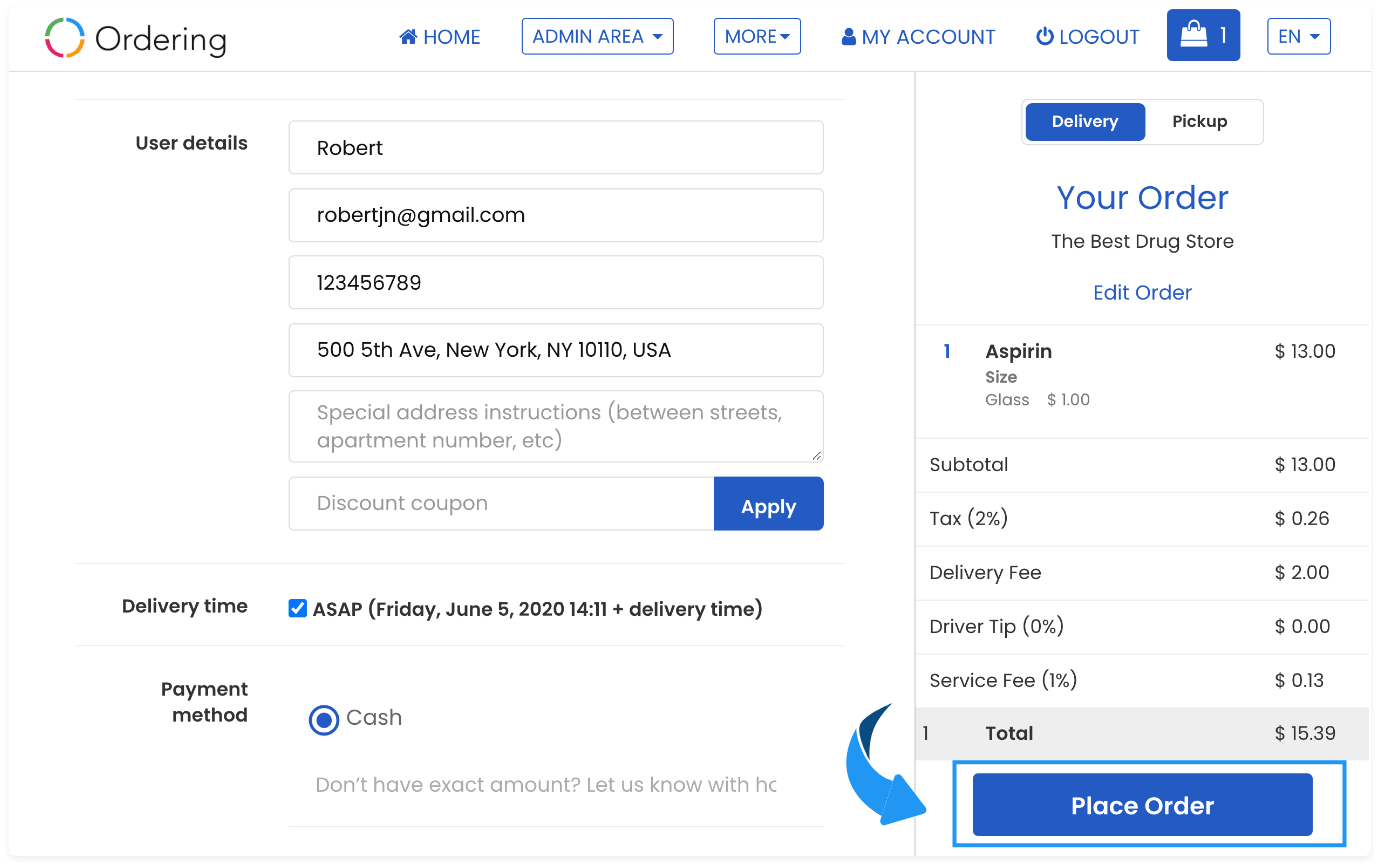Screenshot showing a user interface for an online ordering system. 

**Top Navigation Menu (left to right):**
- "ORDERING" label in the upper left corner.
- "HOME" button with a corresponding home icon in blue text.
- "ADMIN AREA" with a pulldown menu.
- "MORE" with a pulldown menu.
- "MY ACCOUNT" link.
- "LOGOUT" link.
- A blue rectangle featuring a shopping bag icon with the number '1' indicating one item in the cart.

**Main Content:**
- **Form Header**: "USER DETAILS"
- **User Information**: 
  - Name: "ROBERT"
  - Email: "robertjn@gmail.com"
  - Phone Number: "123456789"
  - Address: "500 5th Avenue, New York, New York, 10110 USA"
- **Additional Input Fields**:
  - "Special Address Instructions" (Empty input box)
  - "DISCOUNT COUPON" (Empty input box) with a blue "APPLY" button.

**Delivery and Payment Details:**
- **Delivery Time**: 
  - Method: "ASAP"
  - Date: "Friday, June 5th, 2020"
  - Time: "14:11" plus additional delivery time.
- **Payment Method**: 
  - "CASH"